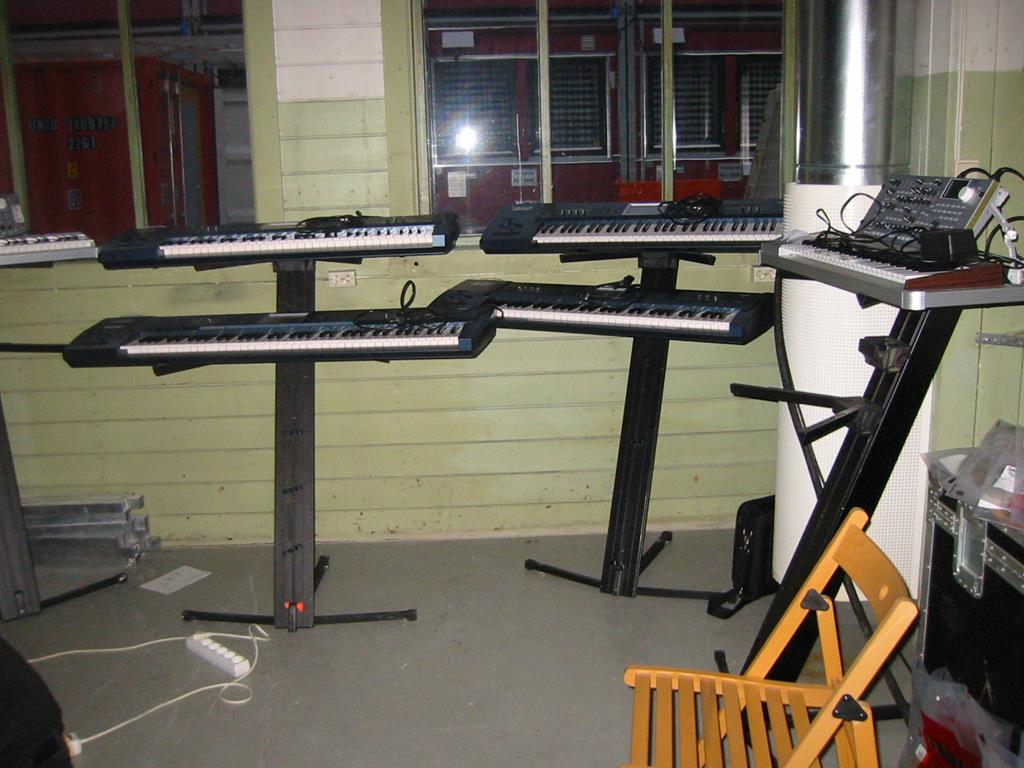The image depicts a spacious, somewhat cluttered music room, possibly in a school or college. The walls are a combination of light green vinyl siding and a very pale off-green paint. There are two wide, sliding windows with light green frames, through which adjacent classrooms can faintly be seen. Along the wall with the windows, there are two stands, each holding two electronic keyboards, making a total of four keyboards on two stands. On the left wall, there is a fifth keyboard with several musical attachments, including a panel with numerous dials and cables, possibly a mixer board. A wooden folding chair with slatted seating is placed randomly in the room. Additional items include a silver-outlined black storage chest, an amplifier on the floor, and an extension cord with multiple plug-ins. The room features a grey floor and appears to be designed for music practice or instruction, albeit in an untidy state.